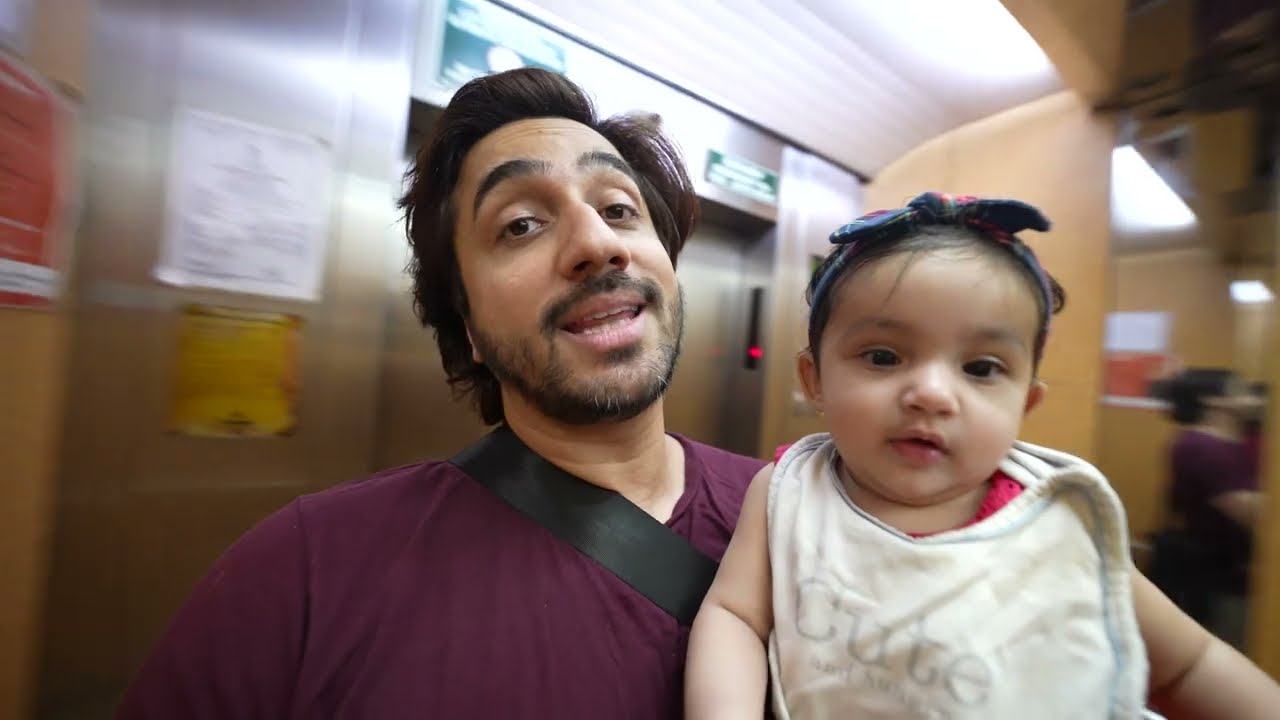In this vibrant photograph, a young father, likely in his late 20s or early 30s, holds his little daughter while taking a selfie. The father has medium to light brown skin, dark eyes, a trimmed black beard and mustache peppered with a few white hairs, and black hair that is either combed back or slightly poofy on top. His eyebrows are raised, and he has an expression as if he’s speaking, with his head tilted back slightly. He is dressed in a plum-colored t-shirt and has a black strap running diagonally across his chest, likely for a bag.

The toddler, presumably a girl around one to one and a half years old, is nestled securely in his arms. She has dark black eyes, wavy black hair adorned with a bow (either blue or black and red), and wears a white bib with the word "cute" printed on it in blue pinstriping.

They appear to be standing in front of elevator doors, which are stainless steel with fluorescent lighting casting a bright glow in the space. The background is slightly blurred, suggesting movement at the time the photo was taken, and there's a hint of a person seated off to the side, adding a sense of depth to the setting.